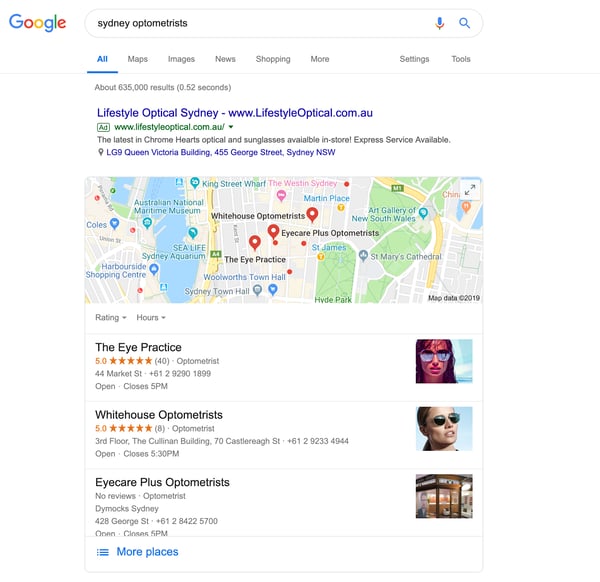The image depicts a Google search results page with a white background. In the upper left corner, the iconic Google logo is displayed, showcasing its distinctive blue, red, yellow, and green color scheme. Adjacent to the logo is the search bar, where the query "Sydney optometrist" has been entered. To the right of the search bar are a microphone icon and a search button.

Below the search bar, various navigation tabs are visible, including "All," "Maps," "Images," "News," "Shopping," and a "More" dropdown option. On the far right of these tabs, "Settings" and "Tools" options are available. The search query has yielded approximately 635,000 results in 0.52 seconds.

The first result listed is for "Lifestyle Optical," followed by "White House Optometrist" and "Eye Care Plus Optometrist."